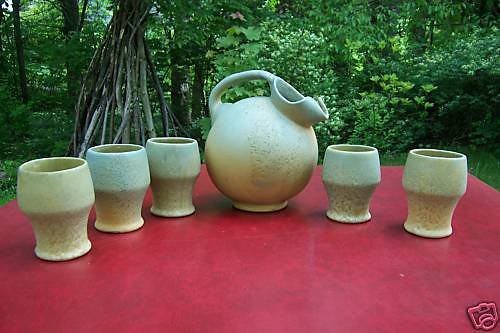This photograph captures an outdoor arrangement of ceramic pottery displayed on a vibrant, mottled red surface. Dominating the backdrop are thin-trunked trees and lush greenery, including light to medium green leaves of various shapes, sizes, and a drooping root system to the left of the frame.

In the bottom right corner, a small red border contains a camera symbol overlay. The pottery is carefully arranged in an arc on the red surface. On the left side, three ceramic cups stand, each slightly wider at the top and narrower at the bottom. In the center, there's a visually striking ceramic pitcher with a large spherical body and an elegant handle that extends across its top, connecting to a uniquely offset spout. To the right of the pitcher, two more ceramic cups similar to the ones on the left make up the display. The overall effect is a harmonious blend of natural and crafted beauty, accentuated by the contrasting bright red background.